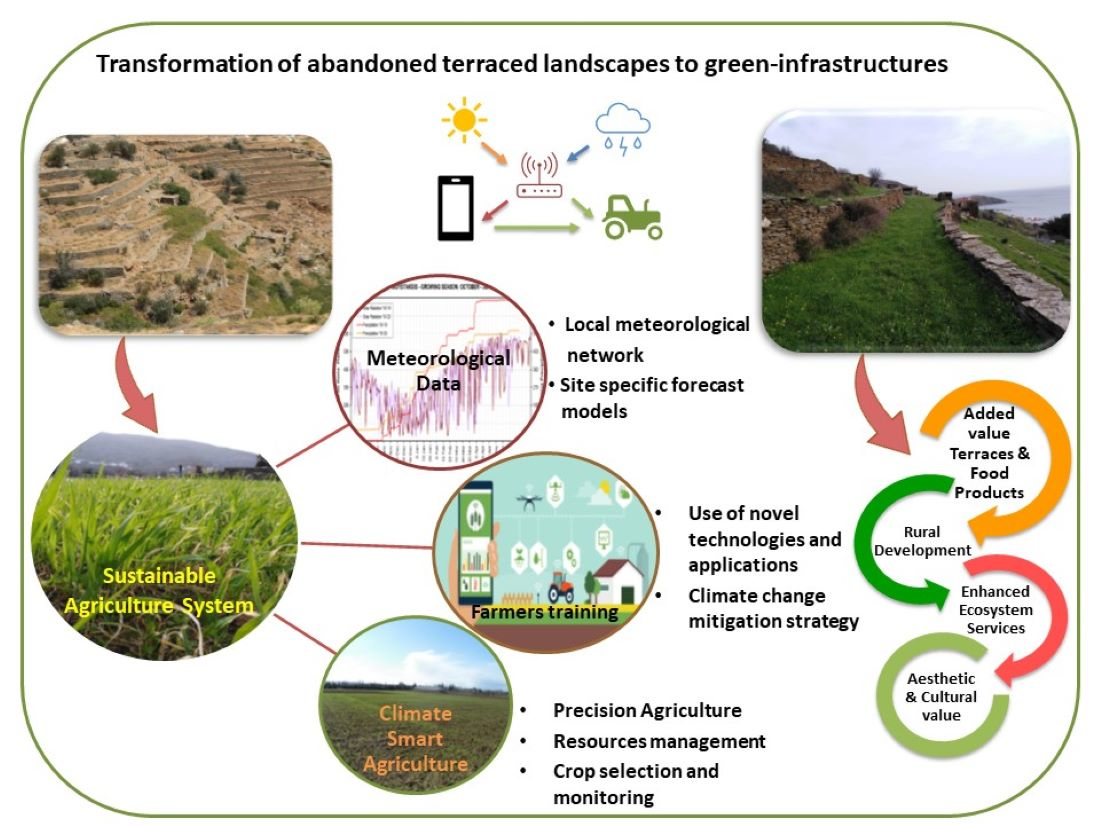The scientific diagram, titled "Transformation of Abandoned Terraced Landscapes to Green Infrastructures," features a detailed and visually organized presentation. The diagram is set against a white background framed by a black border. Central to the design is a rounded square with a clean green line that encompasses several images and diagrams depicting various pieces of landscape transformation.

In the top section, black text reads the diagram's title, emphasizing the transition from abandoned terraced landscapes to sustainable green infrastructures. The left side of the diagram features an image of a brown, sand-like landscape with a tapered stepped formation transitioning into a greener area with stone retaining walls, symbolizing the transformation process. Another image shows vibrant green fields, highlighting the outcome of sustainable practices.

The core of the diagram includes a central focus on a sustainable agricultural system, represented by a prominent circle. From this circle, three lines radiate outward, linking to smaller circles labeled "Meteorological Data," "Farmers Training," and "Climate Smart Agriculture." The "Meteorological Data" circle is detailed with a red circle indicating "local meteorological network" and "site-specific forecast models." Adjacent to this, visual elements depict the integration of modern technology, such as cell phones, drones, and routers, indicating the high-tech aspect of contemporary farming and forestry practices.

Additional details include an icon illustration at the top showing a router with arrows pointing towards a mobile phone and a tractor, accompanied by symbols of sun and rain, emphasizing the importance of meteorological data in agricultural planning. The right-hand side of the diagram shows a rich green hill with stone retaining walls, further exemplifying the landscape's transformation.

Clustered around are multicolored circles (green, orange, red, blue) connected by black text, providing supplementary information on climate-smart agricultural strategies like precision agriculture, resource management, and crop selection. In essence, the diagram conveys a comprehensive overview of transforming neglected landscapes into thriving, sustainable agricultural systems through innovative practices and technologies.